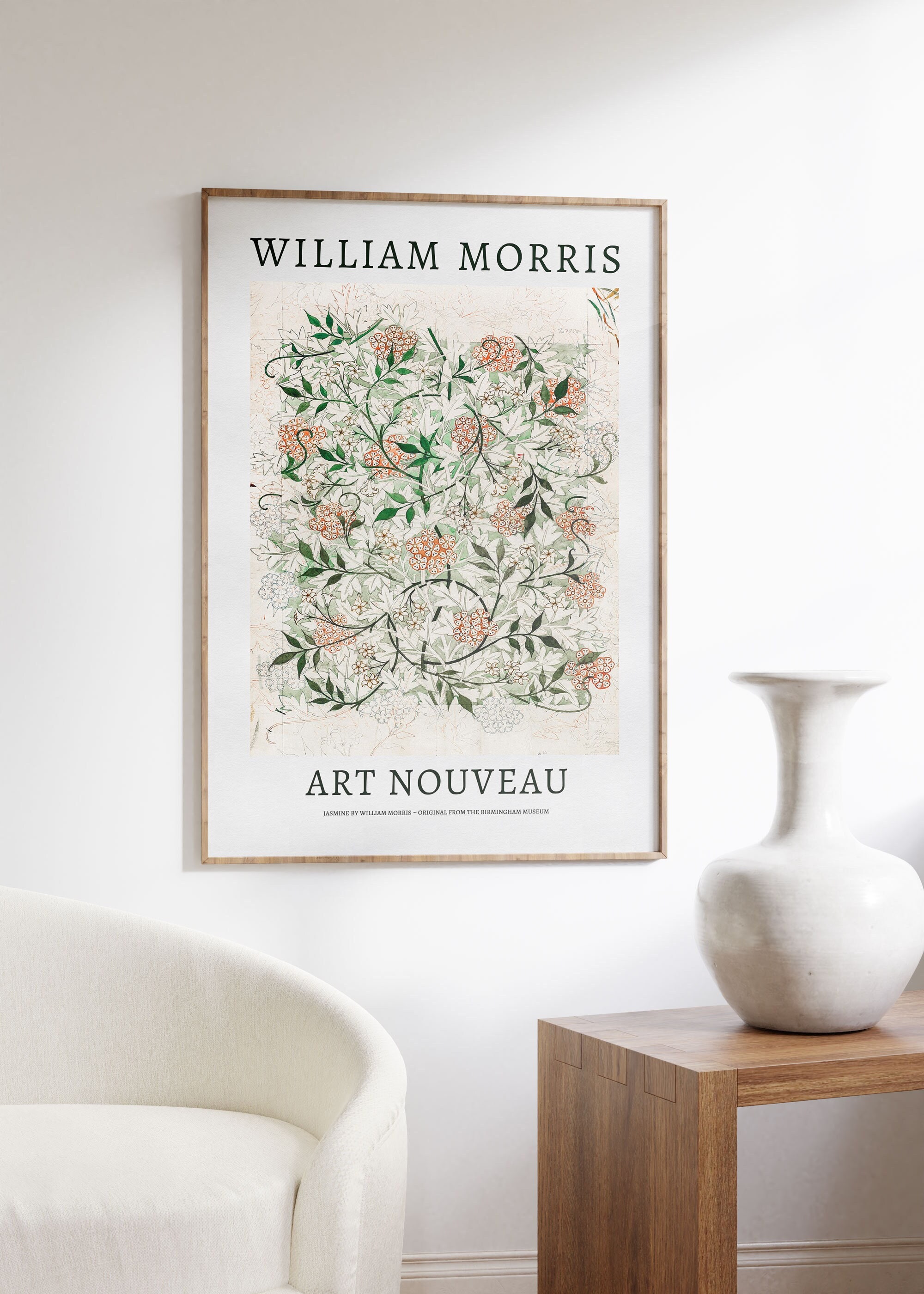The image showcases a beautifully decorated living room. Dominating the cream-colored wall in the background is a framed artwork. The artwork, protected by glass or possibly Perspex, features a delicate rose gold or gold flat metal outline. It prominently displays "William Morris" at the top in thin black text, with "Art Nouveau" at the bottom, and an unreadable smaller sub-line beneath it. The artwork itself is a rich tapestry of spiraling flowers in pale peach and orange hues, interwoven with green leaves, each featuring five leaves and long, curving stems. The background of the artwork is a light yellow shade, complementing the floral design. Positioned in the foreground to the left is a white, curved, padded seat, partially cut off. To the right, there is a sturdy oak side table, designed with interlocking joints, partially in view. Atop the table, a large, exotic white vase with a narrow neck and wide brims at both the top and bottom adds an elegant touch. This well-composed photograph offers a glimpse into an artful and thoughtfully arranged living space.